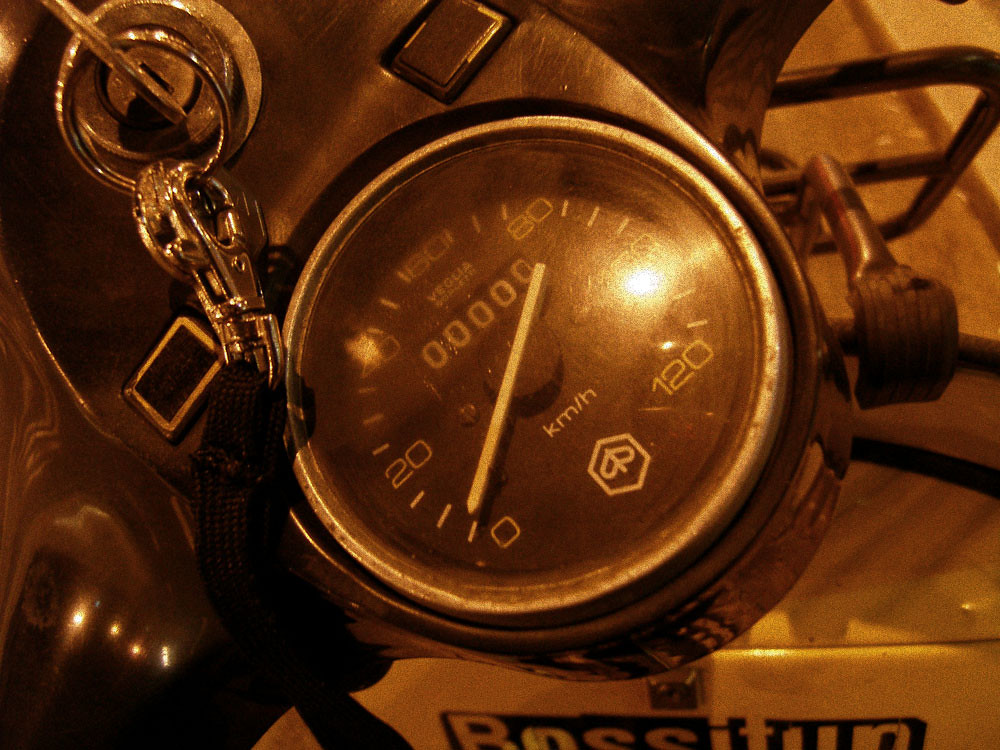A sepia-toned photograph centers on a vintage mechanical doll encased in metal. The doll's face and features appear to be made of glass. Inside the doll, prominently displayed in the center, are the characters "KM-8." A delicate needle rests in the first slot of the central dial, which is intricately marked with numbers from 0 to 120 in increments of 20. To the right of the doll, a key is inserted into a lock, with a fabric strap serving as the key ring. Various metal objects surround the doll, suggesting a mechanical or industrial origin. At the bottom of the image, partly obscured, is the text "BOSSATOM," implying this might be part of an engine, possibly from a lawnmower. The doll is further detailed with metal parts extending in rectangular shapes, adding to the intricate and historical feel of the photograph.